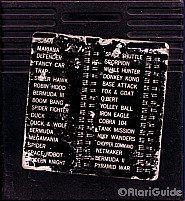The image features a predominantly black background, transitioning from a solid dark upper section. Within this black expanse are elongated, oval-like shapes that almost resemble rectangles at a quick glance, adding a sense of ambiguity to the surface due to the extreme zoom. Occupying the central portion of the image is a large, distressed rectangle that was presumably solid black in its original state. Now, it shows significant wear, with patches of bright white emerging through the black, hinting at previous text that has largely faded. Despite the blurriness that occurs when zooming in, certain words are discernible. On the right side, organized into two columns, fragments of the phrases "base attack" and "goat" are visible. On the opposite side, amidst the distressed markings, the word "car" can be identified, though an adjacent term—which might be "tancy"—remains unclear. Overall, the image presents an enigmatic and textured tableau, marked by the interplay of deteriorated black surfaces and sporadic white text.